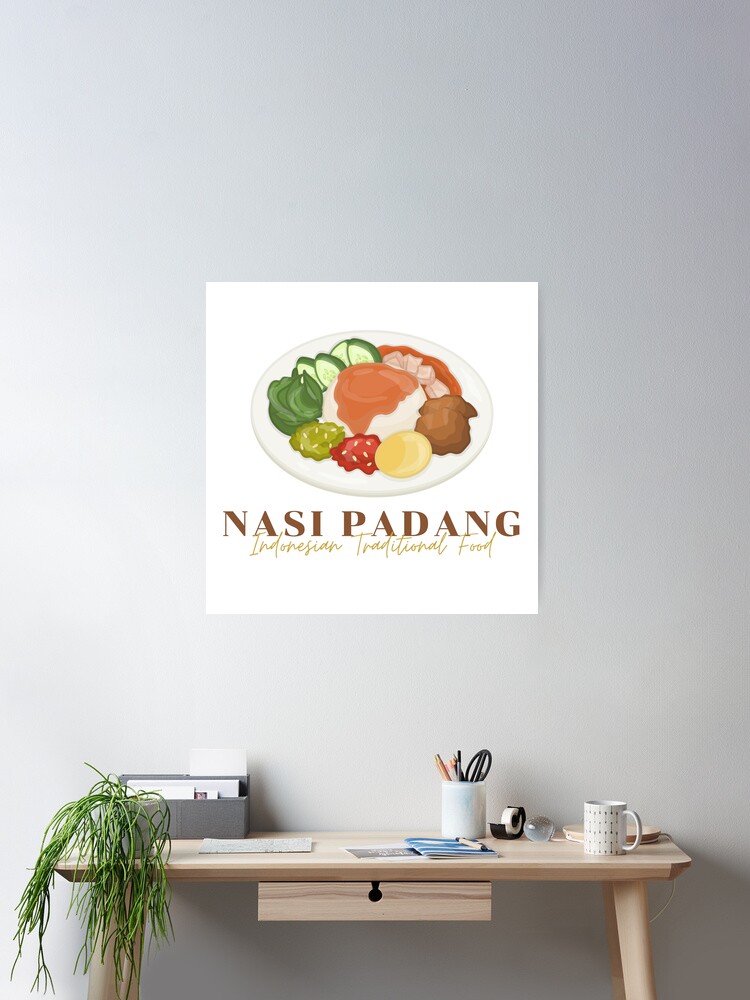The photograph captures a detailed and organized workspace within a room illuminated by soft lighting, giving the white wall behind the desk a slightly dark grey appearance at the top. The focal point of the room is a natural, light wood desk positioned in the lower right corner, with four straight legs extending slightly outward and a rectangular shape. A neat drawer with a small black knob is situated directly underneath the desk surface.

Above the desk on the wall to the left hangs a square poster with a white background featuring a plate of food, including cucumbers, lettuce, ketchup, and an egg, with the words "Nasi Padang, Indonesian traditional food" written in brown. The workspace is adorned with various items: on the left side of the desk sits a green plant and a grey container, while on the right sits a sleek, white desk lamp bending towards the center, a white mug, a roll of tape, and a white pencil holder filled with pencils. This organized and tastefully decorated space appears to depict an office or personal study area.